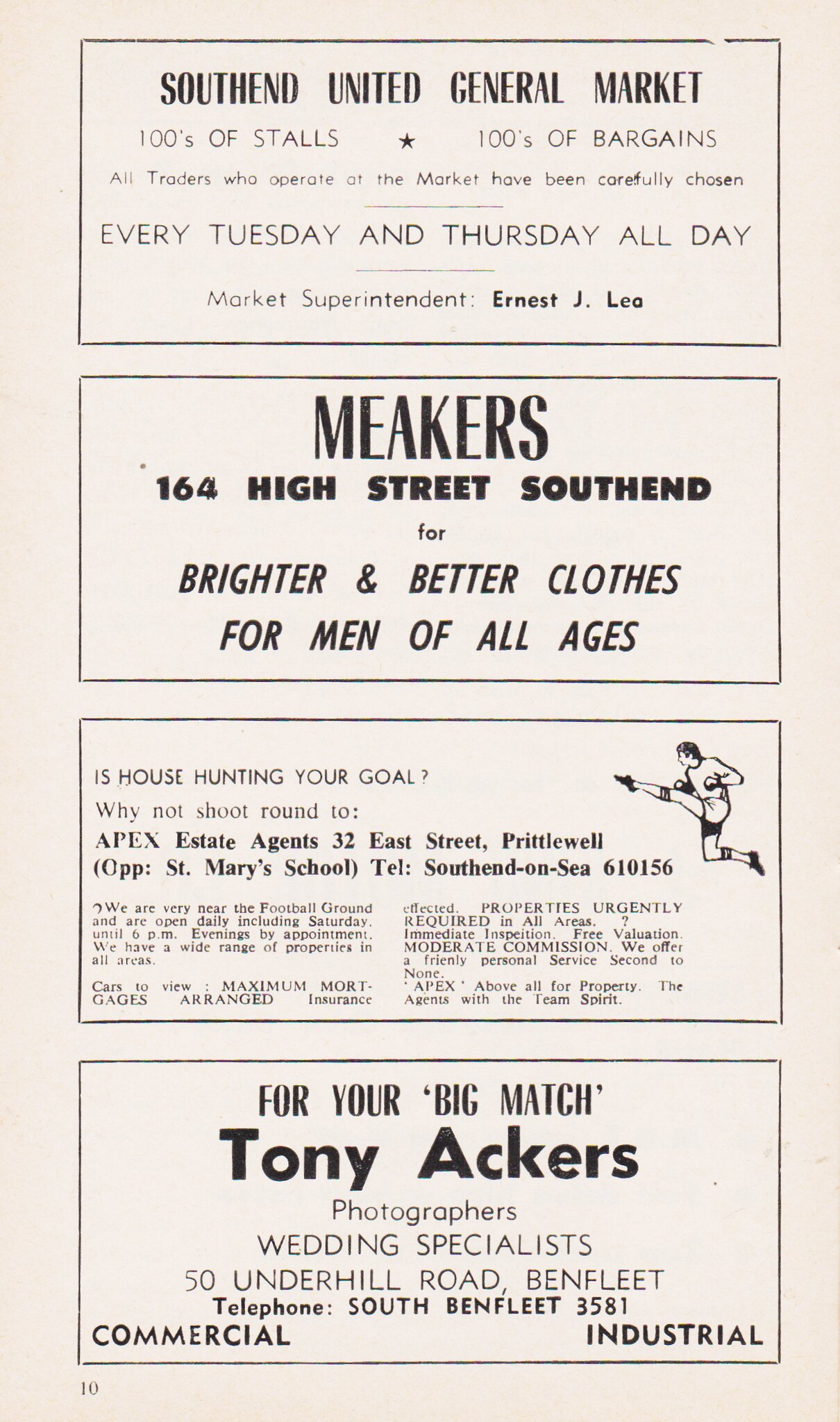This is an old magazine page, possibly page 10 of a larger soccer publication. The page, which has a light pink hue and black ink text, features four rectangular advertisement boxes from top to bottom. The first box promotes the South End United General Market, highlighting "hundreds of stalls, hundreds of bargains" and noting that all traders are carefully chosen. The market operates every Tuesday and Thursday, all day. The second box features Meeker's, located at 164 High Street in South End, offering "brighter and better clothes for men of all ages." A drawing of a soccer player kicking a ball appears in the upper right corner of this box. Below, an ad asks, "Is house hunting your goal? Why not shoot round to Apex Estate Agents," followed by an address for the estate agents. The final box at the bottom advertises Tony Acker's Photographers, specialists in wedding photography, with a listed address and telephone number, noting that they cover commercial and industrial photography as well.